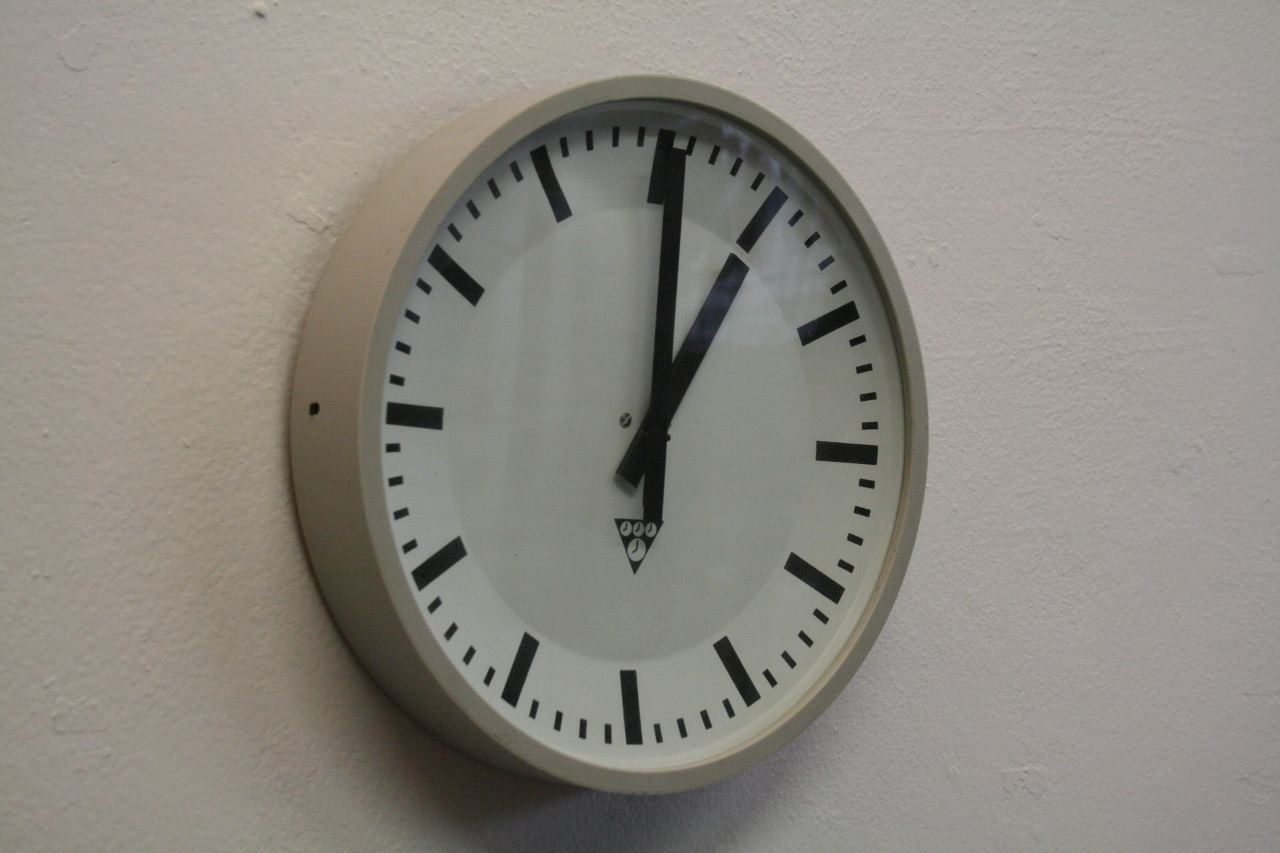This is a color photograph of a clock hanging on a textured white wall. The clock's body is an off-white or light gray color, possibly plastic or metal. The clock face is white and does not have numbers; instead, it features thick black vertical lines at the hour marks and thinner black lines for the minutes. The hands of the clock, which are set to one o'clock, are black, with a longer hand for the minutes and a shorter one for the hours. Beneath the clock hands, there is a distinctive logo resembling an upside-down triangle with small drawings of three or four clocks inside it. A noticeable black mark appears on the left-hand side of the clock's rim. The image does not contain any writing, people, plants, or additional decorative elements, focusing solely on the clock against the white wall.